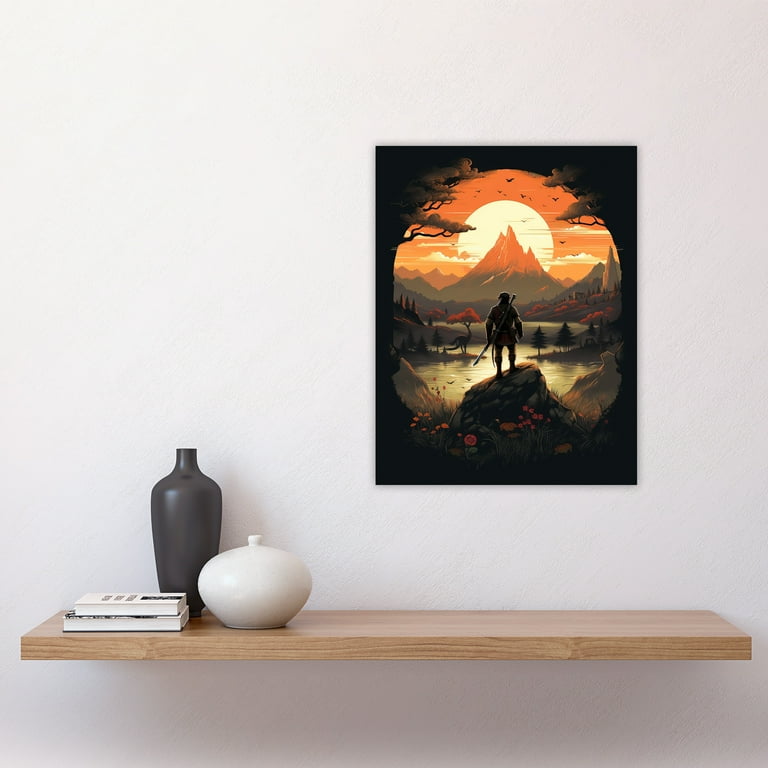This staged photograph, designed in the style of an edited poster for online commercial listings, showcases a visually striking sci-fi fantasy scene. The square-shaped photograph, embellished to appear as though a poster is mounted on a white wall, exudes commercial appeal despite its edited nature, emphasized by the fake shadow behind the flat poster. The central poster, portraying a muscular warrior clad in leather armor with a weapon strapped to his back, captures the viewer's imagination as he stands on a rock. The warrior gazes upon an alien landscape featuring a glowing, orange-hued sunset behind a distant mountain. The scene is dotted with animal-shaped trees, a reflective lake, and a flock of birds soaring in the sky, evoking a strong sense of adventure. Below the poster, a natural wood shelf holds two vases and a pair of books, adding to the stylized, staged composition that effectively highlights the poster as a desirable product for potential buyers.